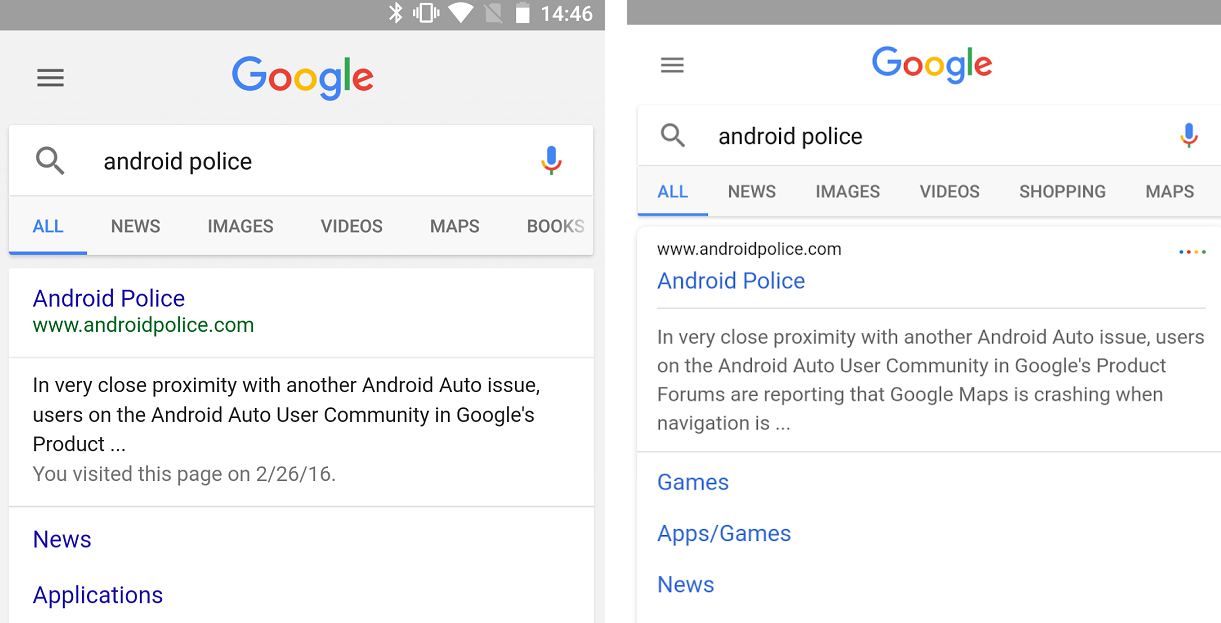The image features two screenshots of Google search results for "Android Police" on different devices. The left screenshot, taken at 14:46, displays a nearly full battery and an active Bluetooth connection. Dominating both screens is the Google logo in its iconic blue, green, red, and yellow colors, accompanied by a magnifying glass icon next to the search query "Android Police."

Both devices feature similar search results but with slight variations in the navigation tabs. The left screenshot includes tabs for "All," "News," "Images," "Videos," "Maps," and "Books." Conversely, the right screenshot replaces "Books" with "Shopping."

In both screenshots, the top search result is a link to the Android Police website. The left screenshot's excerpt reads, "in very close proximity with another Android auto issue, users on the Android user community in Google's product...," with a note that the page was visited on February 26, 2016. Below it, categorized links for "News" and "Applications" appear.

Similarly, the right screenshot features the same top search result, but its excerpt provides a bit more detail: "in very close proximity with another Android auto issue, users on the Android auto user community in Google's product forums are reporting that Google Maps is crashing when navigation is...," followed by links for "Apps," "Games," "Apps & Games," and "News."

All text appears on a white background, with grey for most content and blue for hyperlinks, enhancing clarity and readability.